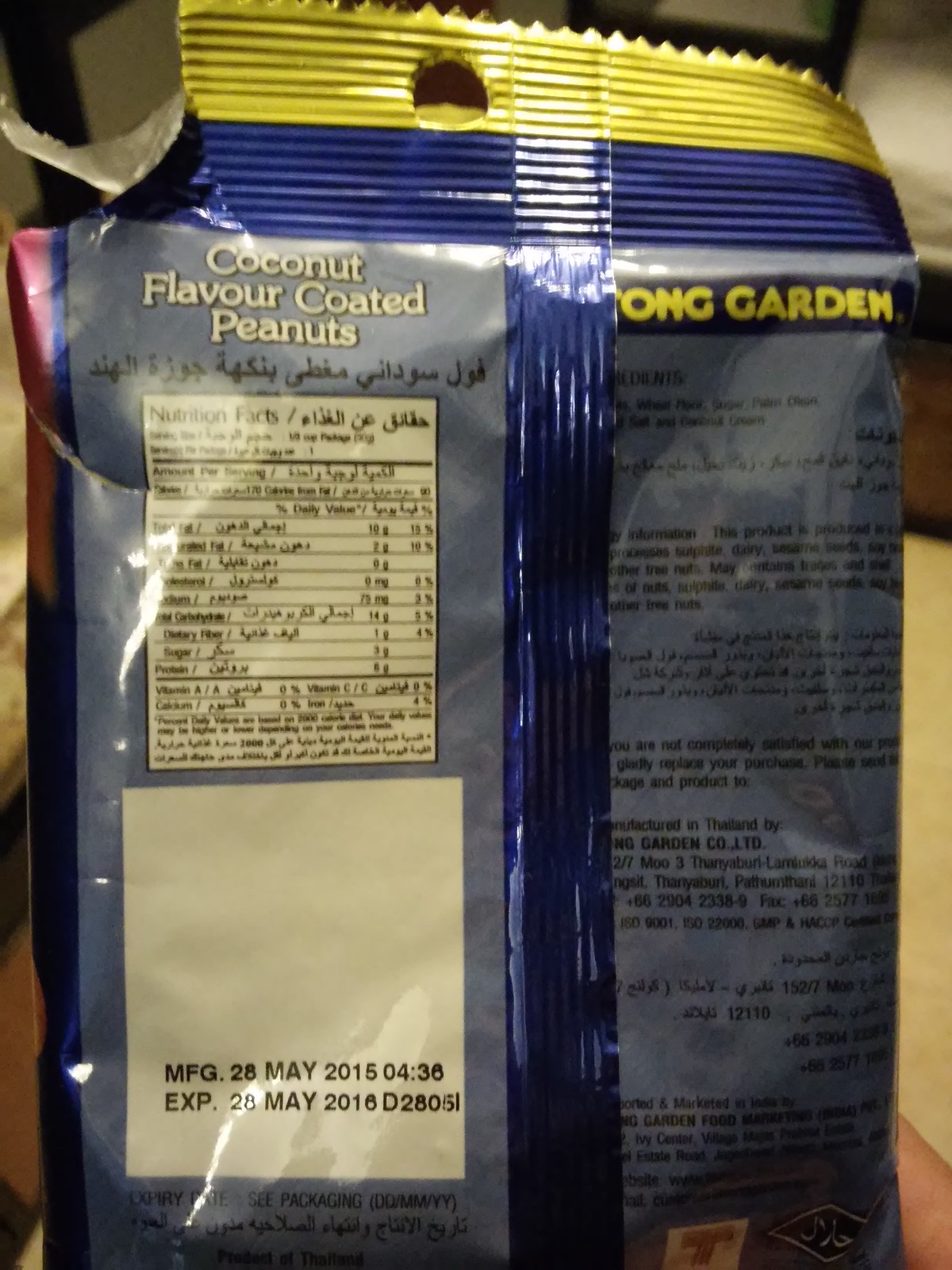This photograph captures the back of a torn plastic package of coconut-flavored coated peanuts. The package features a bright yellow strip at the top with a hole for hanging on a display. Below it, a horizontal dark blue band extends across the package, with a vertical strip of the same blue dividing it into two halves. The background of these halves is a lighter smoky blue. On the left side, the title "Coconut Flavoured Coated Peanuts" is displayed in white lettering, along with a section labeled "Nutrition Facts" in both English and Arabic. This white section stands out against the dark blue. Beneath it, another white box contains black text detailing the manufacturing and expiration dates: "MFG 28 May 2015 04:36" and "EXP 28 May 2016 D28051". On the right side, there is additional black text in Arabic and some indistinct writing, and at the top right corner, partial yellow letters spell out "Something Garden". The package shows a tear at the top left corner, revealing the silver lining inside.